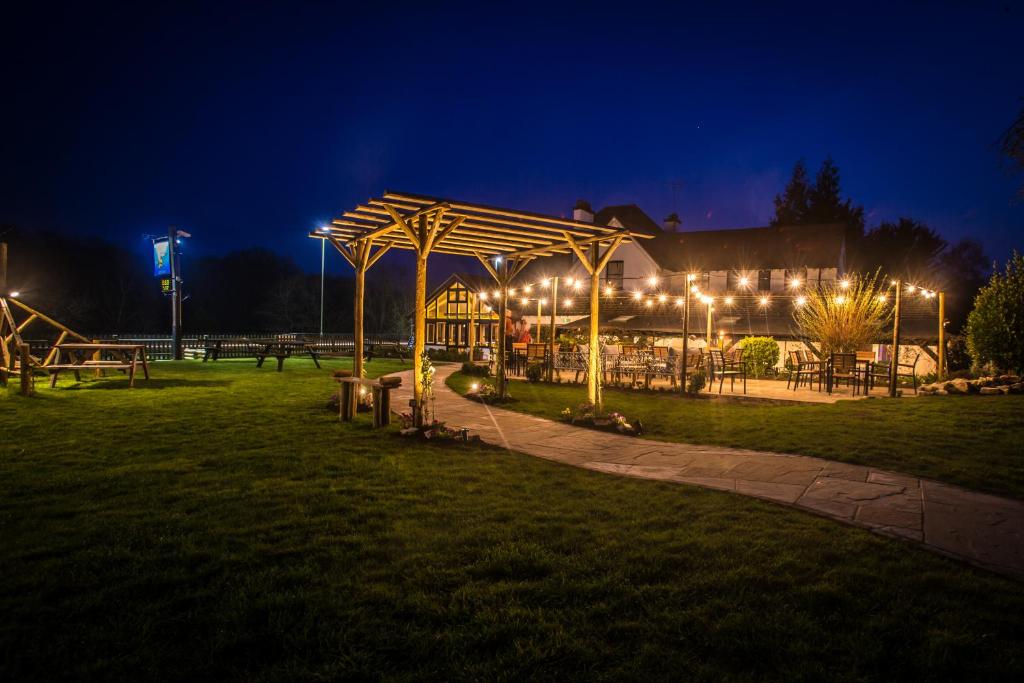This vivid nighttime color photograph captures the enchanting ambiance of a beautiful, possibly European-style residence or restaurant. The photographer is standing in the backyard, showcasing a large and inviting outdoor seating area filled with numerous chairs and tables, adorned with plants and greenery, at the center of the image. A well-lit pathway, paved with cement, winds through the meticulously maintained grass, leading to various picnic tables scattered around. On the left side of the frame, another picnic table is illuminated by soft outdoor lighting. The property is enclosed by a low wooden fence, with trees silhouetted against the striking dark navy blue sky, adding to the picturesque scene. Highlighted in the backyard is a trellis, supported by four logs with horizontal slats, acting as an arbor over the pathway. The entire area is elegantly lit by what appear to be festive string lights, enhancing the serene and welcoming atmosphere.